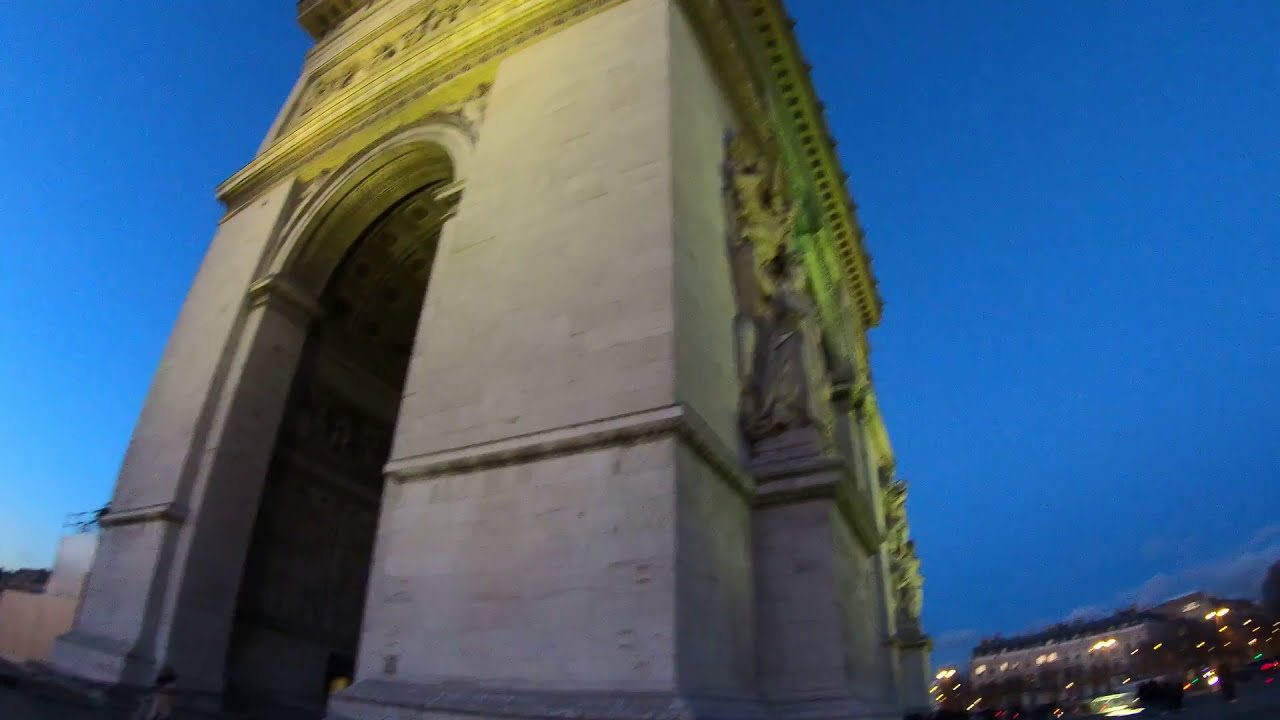The photograph captures a large, classical stone monument reminiscent of the Arc de Triomphe, taken either at dusk or just after sunset. The central feature of the image is a tall, ornate archway constructed from beige stone, adorned with detailed classical fittings and an ornately tiled roof. Statues and sculptures embellish the structure, with notable statues on the right side. The sky is a dark, rich blue, transitioning to lighter hues near the horizon, suggesting the time of day. The image appears somewhat blurred, likely due to motion, possibly from being taken inside a moving vehicle, which also affects the illuminated background buildings, giving them a slightly hazy appearance. The archway stands prominently, its height estimated between 20 to 30 feet, evoking historical edifices through which troops might have marched in Roman times.